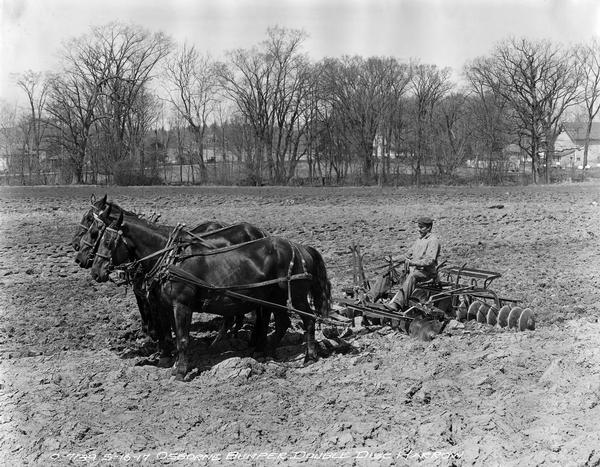In this evocative black and white photograph from the 1950s or 60s, a farmer is seen tilling his dry, parched land, preparing it for planting. Seated on an antiquated, metallic plow designed to make divots in the soil, the farmer holds the reins of three powerful black horses that pull the apparatus. The plow, adorned with circular discs at the back, is being skillfully maneuvered to mix the dirt and ready the field for seeds. Background elements include a grey sky, leafless trees, and a row of houses, all contributing to the nostalgic agrarian setting. The picture captures the essence of traditional farming practices with a backdrop of natural and rural elements.